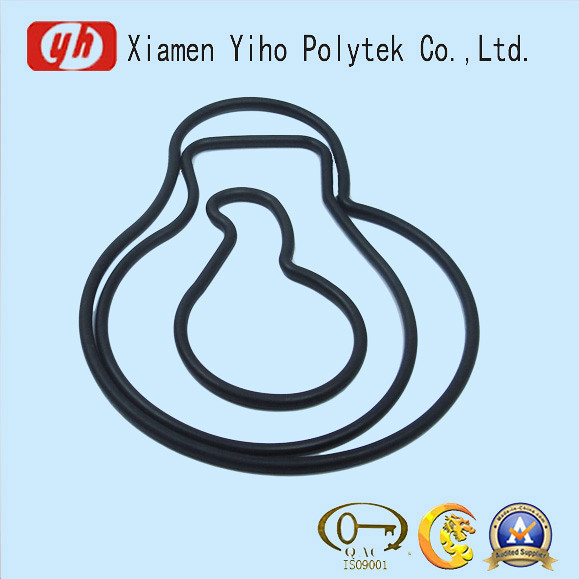This image appears to be a digital advertisement likely for a company that produces ropes or fibers, set against a pale blue background. The layout is more vertical than horizontal, dominated centrally by black, rubbery rope-like outlines that form a nested series of pear-shaped designs. In the upper left corner, there’s a red logo with the letters "YH" and black text adjacent to it that reads "Xiamen Yeho Polytech Co. Ltd." Below this, slightly more to the middle, are the interconnected black outlines resembling pears, which stand out against the light blue backdrop. In the bottom right corner, three logos are aligned from left to right: a gold key, a dragon also in gold with a tail forming a C-shape, and an 'A' with a checkmark within a gold-bordered blue circle that reads "Audited Supplier". The image's elements suggest a focus on branding and certification, conveying the company's identity and credentials effectively.